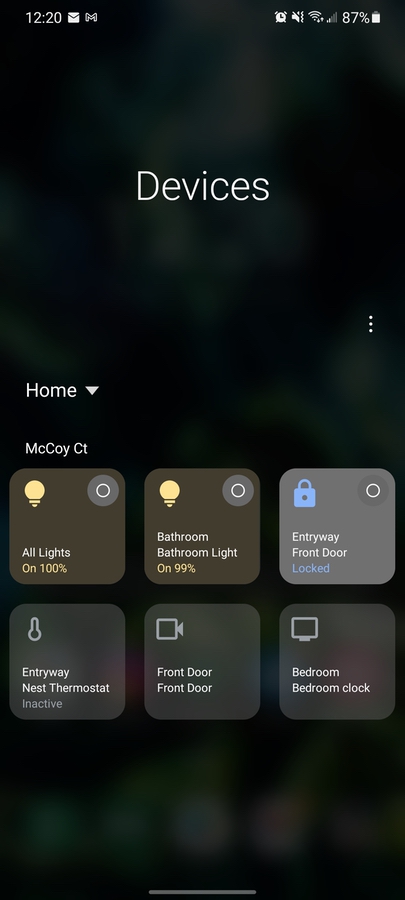In this image, a smartphone displays a home automation app with a dark background and various status icons at the top of the screen. The time reads 12:20, accompanied by an email icon and a Gmail icon. At the top right, there are icons indicating a battery level of 87%, network status, Wi-Fi connectivity, and an active mute and alarm.

The app interface features a header that reads "Devices in Height." Directly below, on the left side, there's a dropdown option labeled "Home," and on the right are three vertical dots indicating additional menu options.

The main interface of the app is organized into a grid of six buttons. The first button, titled "All Lights On 100%," has a brown background with a yellow light bulb icon. Next, the "Bathroom Lights On 99%" button also features a yellow light bulb on a brown background. The third button reads "Entryway Front Door Locked," and is accompanied by a blue lock icon.

On the bottom row, the first button states "Entryway Nest Thermostat Inactive" with a grey background. Beside it, "Front Door" is displayed with a video camera icon. The last button is labeled "Bedroom Clock" and features an icon of a smart device.

This app allows users to control various home devices, including lights, locks, thermostats, and more, from their smartphone.